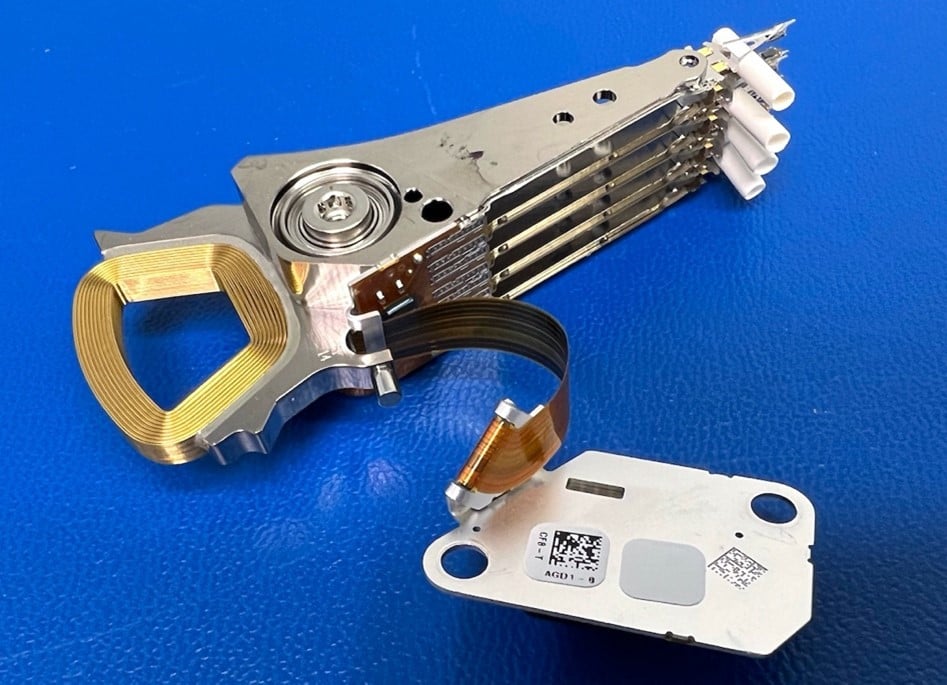The image depicts a perplexing, silver-toned mechanical device set against a medium blue, pebbly-textured background. Central to the image is a roughly triangular, stainless steel or aluminum object. On the right-hand side, this object features four horizontal rows, each protruding with small, white, cylinder-shaped tubes. To the left, there is a handle-like opening lined with a gold or bronze trim. Emerging from the bottom of this handle section is a black band or tape material, connecting to a separate, flat silver plate. This attached plate, presumed to be metallic and chrome-colored, has two circular holes at its opposing corners and is marked with two QR code stickers. The device's overall appearance suggests a piece of electronic machinery or equipment, though its exact purpose remains ambiguous.